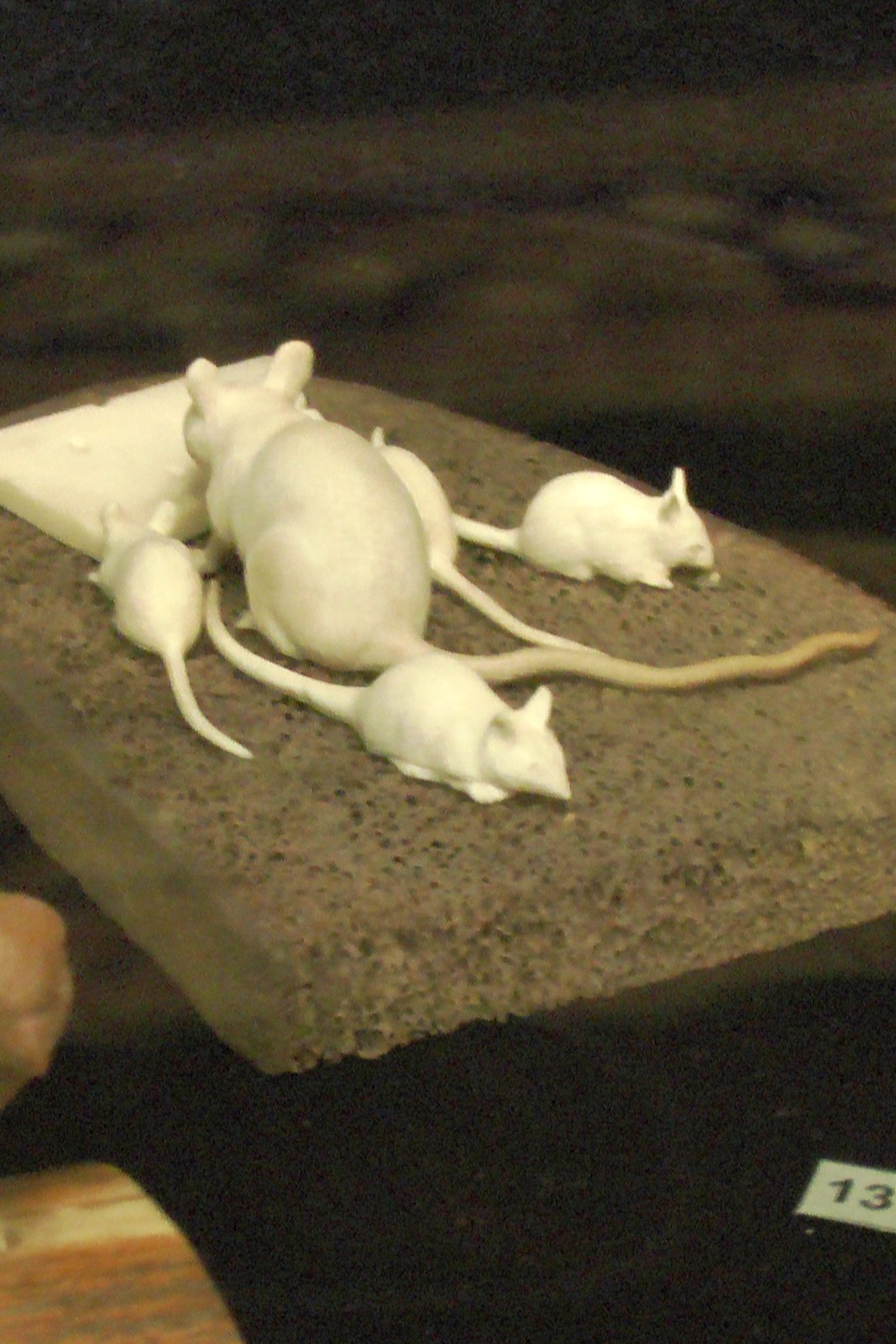The image depicts an intricate artistic sculpture featuring a mother rat and her four baby rats, all crafted from white clay or porcelain. The mother and two of the baby rats are depicted nibbling on a slice of white clay cheese, complete with detailed dents. The three other rats have their backs turned, seemingly exploring their surroundings. All the rats have elongated tails, adding to the realism of the artwork. They are positioned on a grayish speckled base that appears to be made of either a wooden plank or a granite slab. In the background, a blurred floral patterned carpet is visible along with what might be a brick wall. The lower right corner of the base is marked with the number 13, suggesting it may be part of an exhibition or a series. Subtle details such as potentially visible hands and a wooden structure to the left enhance the depth and context of the scene.